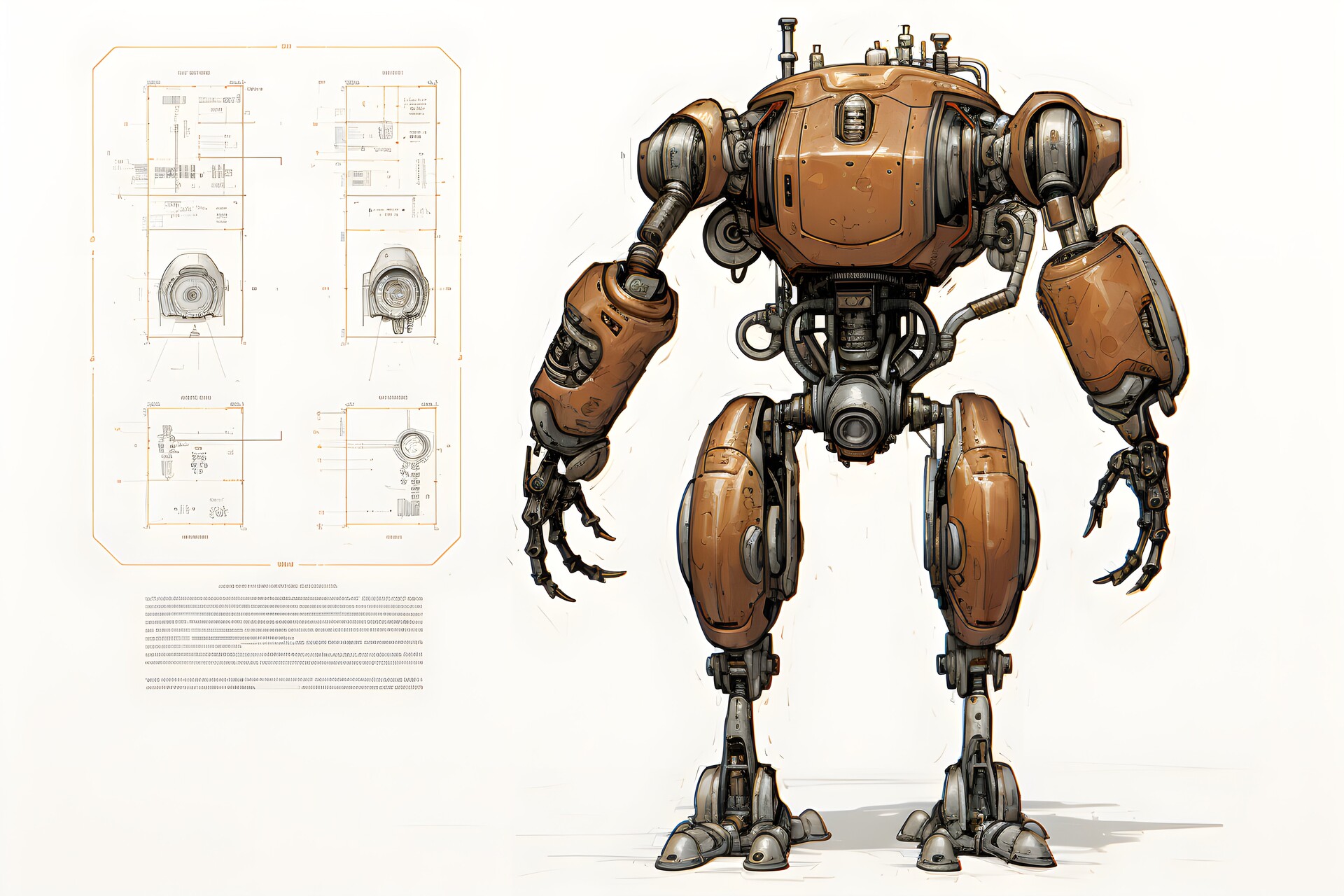The image is an elaborate illustration of a headless robot resembling those found in science fiction fantasy shows or a Star Wars movie set. The robot stands upright on the right-hand side, showcasing a copper brown and gunmetal gray color palette. Its chest plate, forearms, and thighs are brown, while the shoulders, feet, and claw-like hands are metallic silver. The feet are described as bulky and chicken-like, suggesting both strength and agility, while the hands, eerily equipped with three pointed fingers and a thumb, enhance its menacing appearance. On top of its body, small screws and pipes are visible, adding to the intricate detail. Notably, there is an object resembling a telescope emerging from the area where its genitalia would be. To the left of the main illustration, there is an exploded diagram, presumably detailing the robot's cameras, sensors, or other components, although the small print renders the annotations unreadable. Underneath this schematic, paragraphs of text further explain the diagram, but like the annotations, the text is too diminutive to decipher.